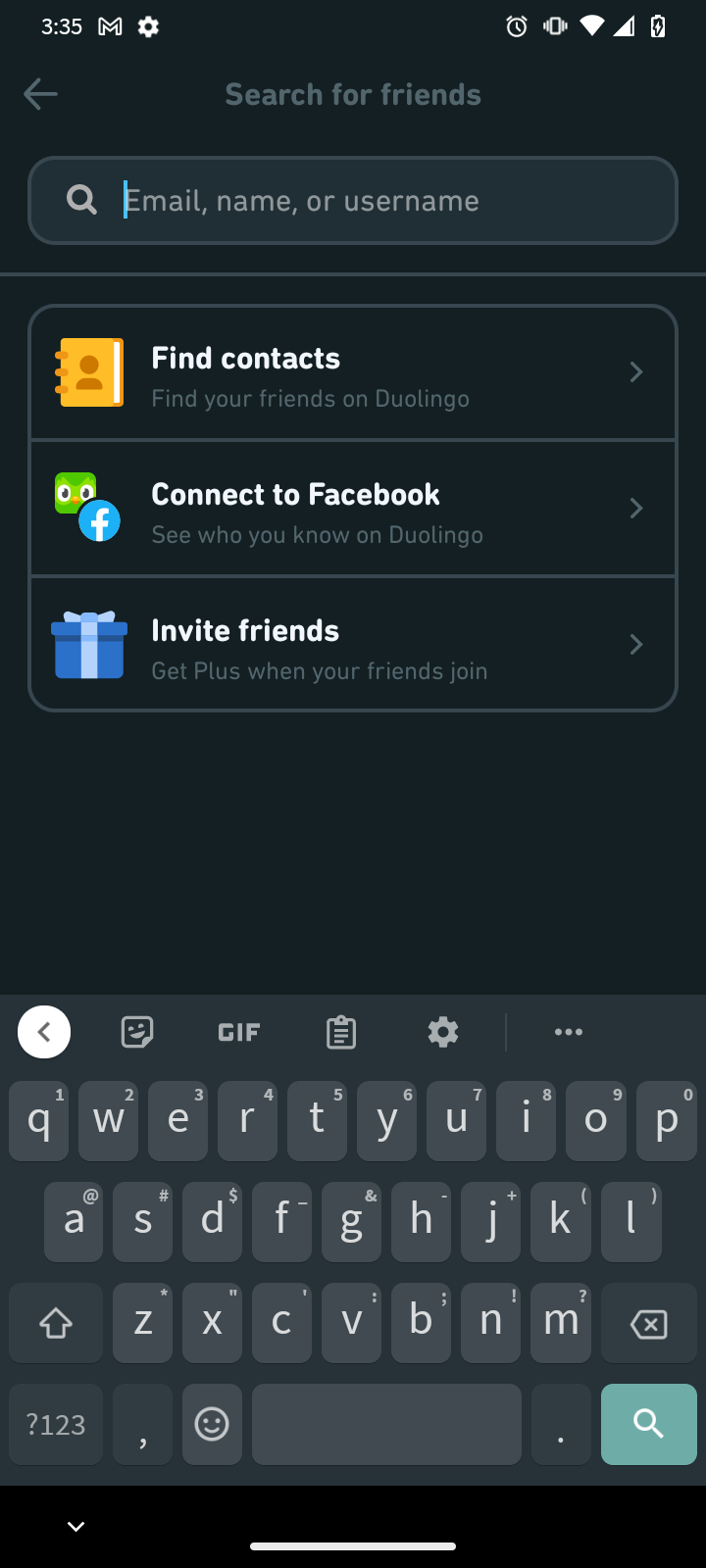A detailed screenshot of a mobile phone features a predominantly black background. The top left corner displays the time “3:35,” followed by a gear icon. To the right, a clock icon, a Wi-Fi signal indicator, and a battery icon are visible. Below this status bar is a search bar labeled “Search for Friends.”

Underneath the heading "Search for Friends," a text input field with the placeholder “Email, name, or username” is accompanied by a search icon on the left.

The screenshot then transitions into a black section containing three horizontally-aligned options. The first option, illustrated with a book icon, reads “Find Contacts - find your friends on Duolingo.” The second option, marked by both the Facebook and Duolingo icons, states “Connect to Facebook - see who you know on Duolingo.” The third and final option, denoted by a blue present icon, says “Invite Friends - get Plus when your friends join.”

Below these options, another black area precedes a QWERTY keyboard that has popped up at the bottom of the screen for user input.